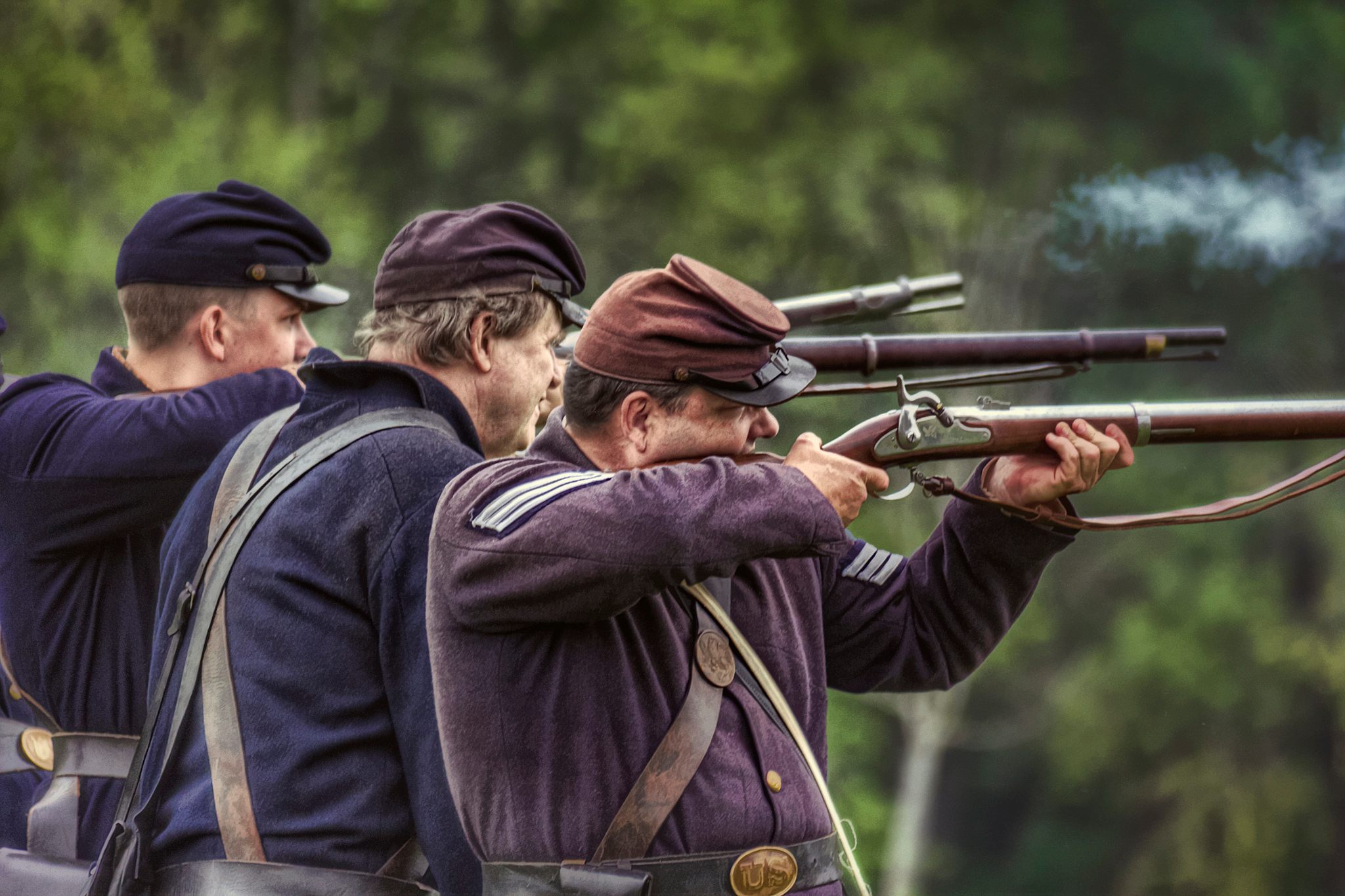The image showcases a detailed scene of a historical battle reenactment with three men dressed in period attire. The central figure, who is prominently positioned with his torso slightly twisted toward the viewer but looking to the right, is holding a musket or rifle—likely a flintlock given its old-fashioned firing mechanism. He is garbed in a dark purplish coat, a reddish hat, and gray pants. Behind him, two additional figures are aligned; they are similarly attired in long blue shirts tucked into gray pants, and they also wear styled hats that are small-visored, bunching slightly at the front. All three men appear to have utility straps across their shirts and are in the act of firing their weapons, evidenced by the visible smoke around them. The scene is set against a backdrop of green trees, enhancing the historical atmosphere of the reenactment.